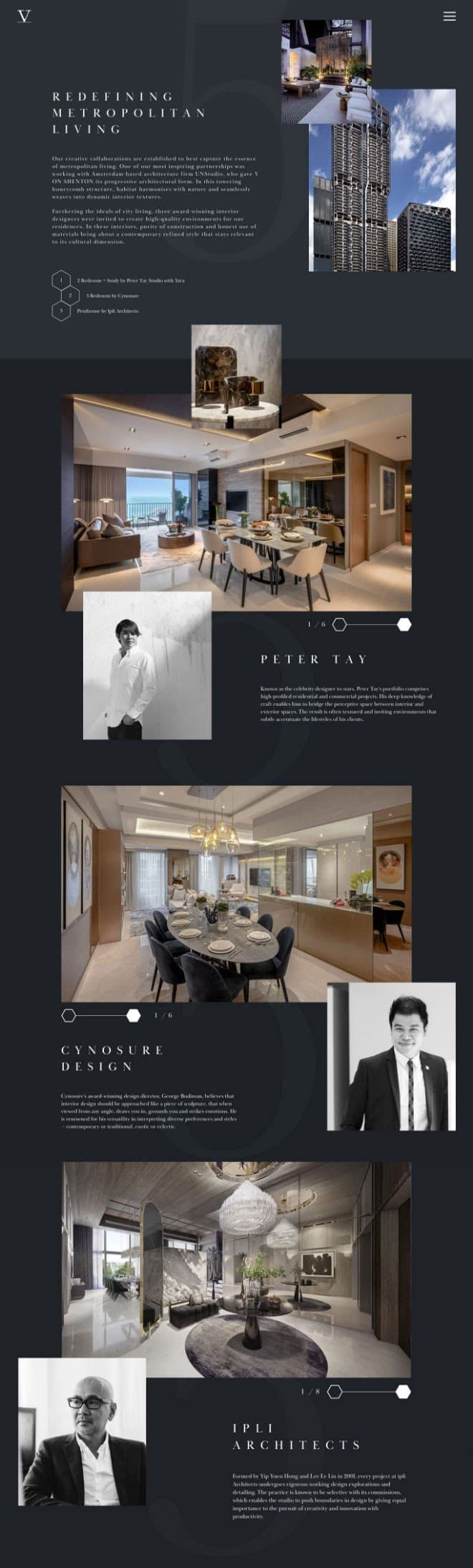**Caption: A Glimpse into Metropolitan Elegance and Design Innovation**

The image provides a detailed look into a concept that redefines metropolitan living. The visual presentation has been skewed for maximum informational content, which unfortunately makes it difficult to read the text clearly. The prominent heading "Redefining Metropolitan Living" stands out against a black background with white font. 

Embedded within the design, three honeycomb-shaped octagons add an abstract artistic touch. The small, skewed text within these shapes remains unreadable. Two primary photographs showcase striking views, one seemingly depicting the exterior of a modern high-rise building and another hinting at an interior space within such a high-rise.

Additional images beneath these highlight chic interiors—possibly of a restaurant, given the multitude of dining tables arranged elegantly. The name "Peter Tay" is mentioned, suggesting his involvement in the design, though specific details about him are illegible. A photograph, likely of Peter Tay, accompanies this section.

Further down, more images reveal an expansive dining table, aligning with the sophisticated restaurant theme. The label "CYNOSUR Design" appears, albeit with unreadable accompanying text. Another individual is featured in a photograph below this, yet without further identifiable context.

Finally, the label "IPLI Architects" along with another portrait, presumably of an architect affiliated with the firm, concludes the visual narrative. The overall image exudes a sophisticated, metropolitan aesthetic intertwined with modern architectural and interior design principles, despite the challenges imposed by the distorted text visibility.